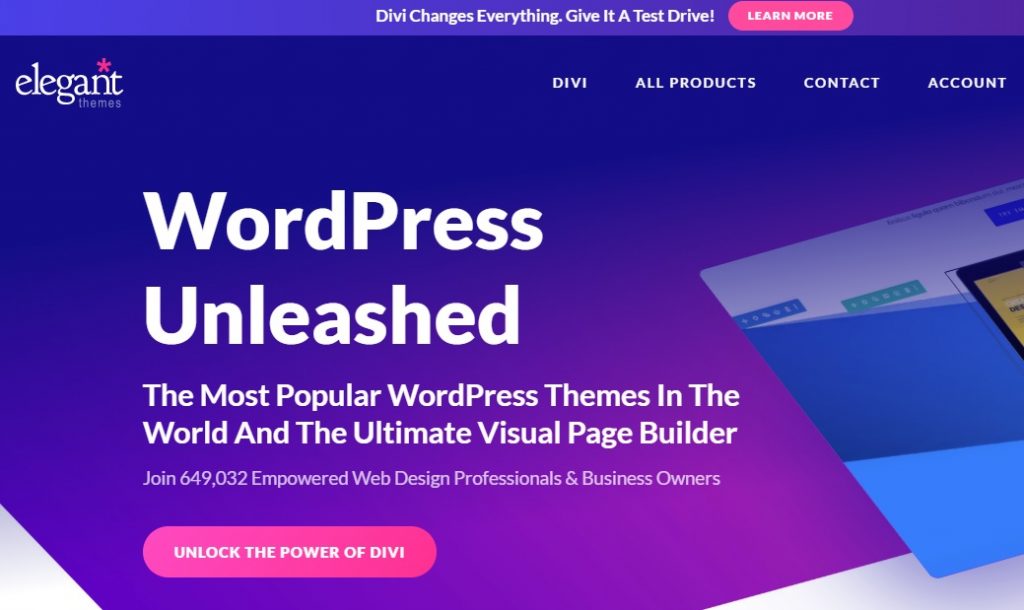At the very top of the image, a long purple rectangle prominently displays white text that reads: "DIVI changes everything. Give it a test drive!" To the right of this text, inside a red circle, the words "Learn More" are highlighted. 

In the lower-left corner of the image, the company name "elegant" appears in lowercase letters, with a red star positioned above the letter "N". Moving to the right of this, the navigation options include "DIVI," "All Products," "Contact," and "Account."

The background at the top of the image is a deep purple, which gradually transitions to a lighter purple as it descends. Centered in this gradient background, the main text in white reads: "WordPress Unleashed." Below this, an explanatory text states: "The most popular WordPress themes in the world, and the ultimate visual page builder."

Further down, bold purple text encourages readers to "Join 649,032 empowered web design professionals and business owners."

At the bottom of the image, a long, pill-shaped button in white uppercase text invites action with the words: "UNLOCK THE POWER OF DIVI."